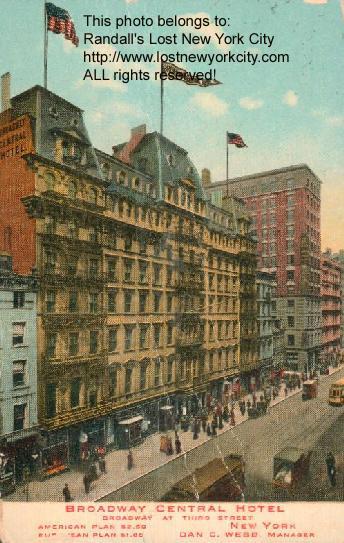This vintage promotional image for the Broadway Central Hotel, appearing like a watercolor or early photorealistic artwork, showcases a partially frayed and rough depiction of New York City from the 1920s or 1930s. Dominating the center, the hotel stands tall within a city block, featuring a yellowish-brown facade adorned with three distinct fire escapes. Above the building, a clear blue sky is decorated with two American flags on either side and a pennant in the center. The hustle and bustle of city life enliven the scene below, with people walking on the sidewalks and streetcars and other early 20th-century conveyances moving along the road. At the top of the image, digitally superimposed text reads, "This photo belongs to Randall's Lost New York City, www.lostnewyorkcity.com, all rights reserved," against the sky. The bottom of the image, bordered in white, bears bold red lettering that says "Broadway Central Hotel," followed by smaller, somewhat blurry text providing additional details about the hotel's address and location.